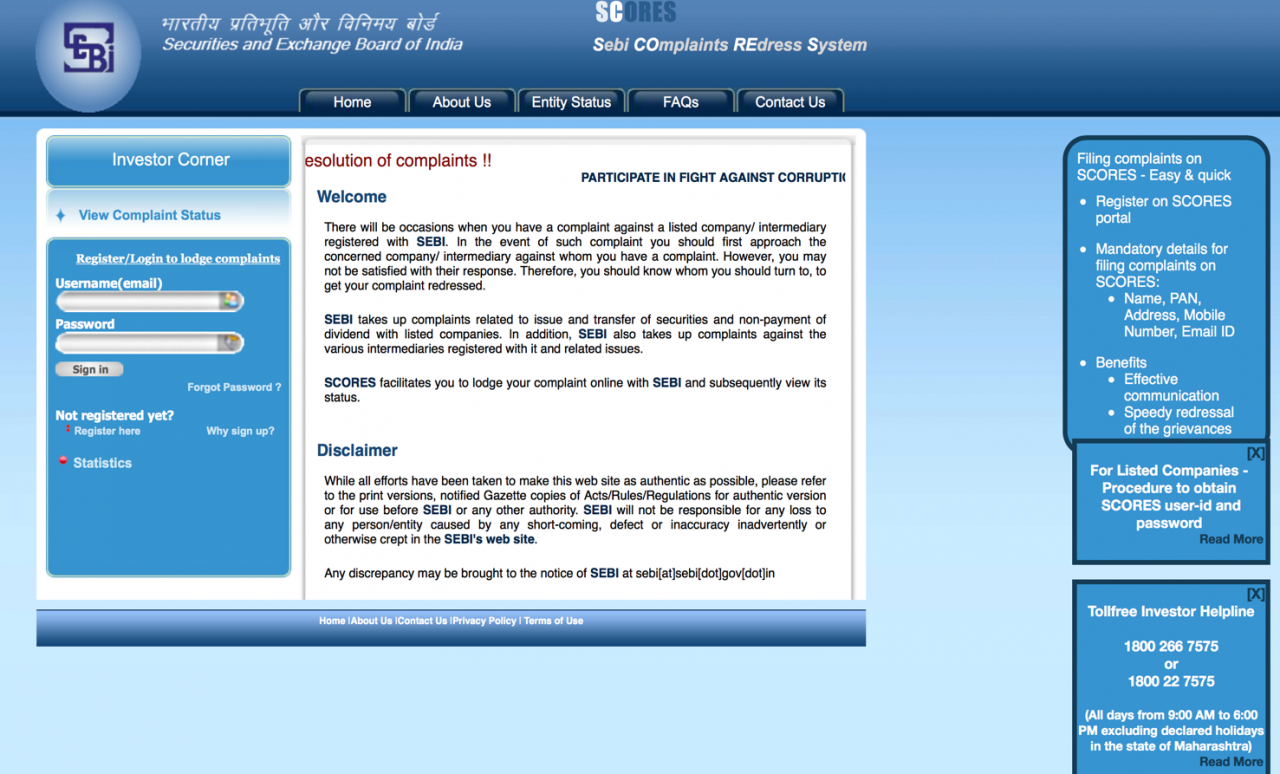The image features a light blue background with various sections in different shades of blue and white. At the top of the image, there is a slightly darker blue box that contains a light blue circle with the letters "C" and "B" intersected by a large "S." This emblem is accompanied by white text in a foreign language. Below this emblem, the text "Securities and Exchange Board of India" is prominently displayed.

Further down, the word "SCORES" is shown with "SC" in white and "ORS" in blue, followed by the subtitle "SEBI Complaints Redress System." Below this title, there are several navigation tabs labeled "Home," "About Us," "Entity Status," "FAQ," and "Contact Us."

Underneath these tabs is a white box with a blue header titled "Investor Corner," featuring options such as "View Complaint Status & Register" and "Log In to Lodge Complaints." It includes fields for "Username" and "Password" as well as "Sign In" buttons. There are also instructions for users who are "Not Registered Yet."

A larger section of the image is dedicated to "Resolution of Complaints & Participate in Fight Against Corruption," which includes a welcome message and disclaimer. At the bottom of this larger section, there is a blue box with white text.

To the right side of the image, there are three small blue boxes. The first box highlights that "Filing Complaints on SCORES is Easy and Quick" with step-by-step instructions. The second box is directed at "Listed Companies" and elaborates on the procedures to obtain SCORES, User ID, and password, with a "Read More" link in blue. The third box provides information on the "Toll-Free Investor Helpline" along with the helpline number and another "Read More" link at the bottom.